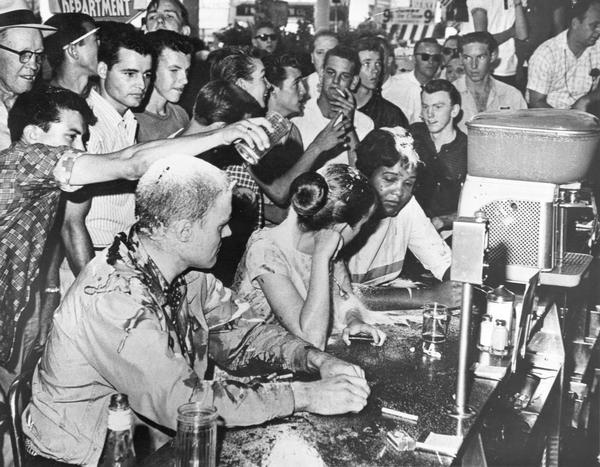The black and white photo, likely taken in the 1950s or early 60s, captures a tense moment of apparent harassment at a classic diner or bar. Three individuals, two women—one notably with a distinctive white stripe in her black hair—and a man with short hair, are seated at a counter. Their clothes are visibly drenched, indicating they’ve had beverages poured over their heads, with liquid spilling onto the counter. The man appears to have wet sleeves and collar, emphasizing the mess created. Behind them, a crowd of mainly men, some smoking or with cigarettes tucked behind ears, looms ominously. One man in the background is caught mid-act, about to pour a drink over the head of the woman with a bun. The bar is detailed with everyday items such as a beer tap, salt and pepper shakers, and a juice machine, grounding the scene in its time period. The overall atmosphere hints at an act of public humiliation, set against a backdrop of potential racial tension.